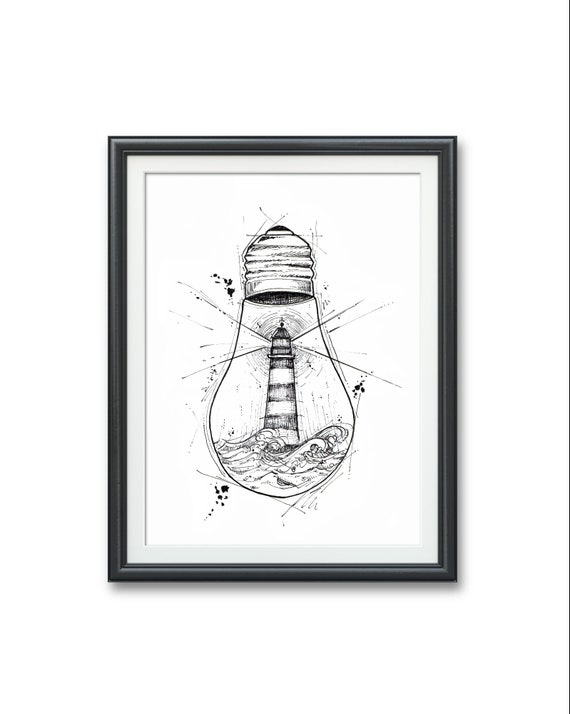The image is a detailed sketch that depicts a creative juxtaposition of a lighthouse inside an upside-down lightbulb. Done in a style that could be pencil, charcoal, or pen, the lighthouse features alternating black and white stripes and sits on a small ocean with visible waves curling up beneath it. Rays of light emanate from the top of the lighthouse, extending beyond the confines of the bulb. This intricate drawing is set against a white background, bordered by a white mat and encased in a black frame, all hung on a white wall. The sketch has a meticulously detailed, slightly sketchy quality that suggests an expressive, exaggerated etching technique, emphasizing the lighthouse's striking light and the surrounding waves. The entire composition blends seamlessly into its monochrome presentation, highlighting the high level of attention to detail and the cleverness of the artwork's concept.